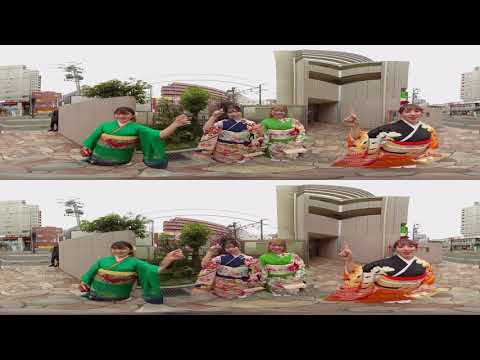The image showcases four women dressed in elaborate traditional Japanese clothing, standing on a cobblestone street in an outdoor urban setting. The woman on the far left is wearing a green kimono with a red sash and a yellowish stripe, and she holds her left hand upright, almost in the shape of a fist. Next to her, the second woman dons a kimono featuring a blue chest area with predominantly white, red, and pink on the sleeves and lower torso. The third woman’s kimono is primarily green in the center, accented with white, yellow, and red hues on the rest of the garment. The woman on the far right is clad in a kimono with a navy blue or black shoulder area and the rest mainly in red and orange. They appear to be standing in front of a large gray structure, possibly the entrance to a subway, with trees and various buildings visible in the background. The image is duplicated and stacked horizontally, showing the same scene twice from left to right. The women are smiling and gesturing towards the camera, contributing to the vibrant and cheerful atmosphere of the picture.